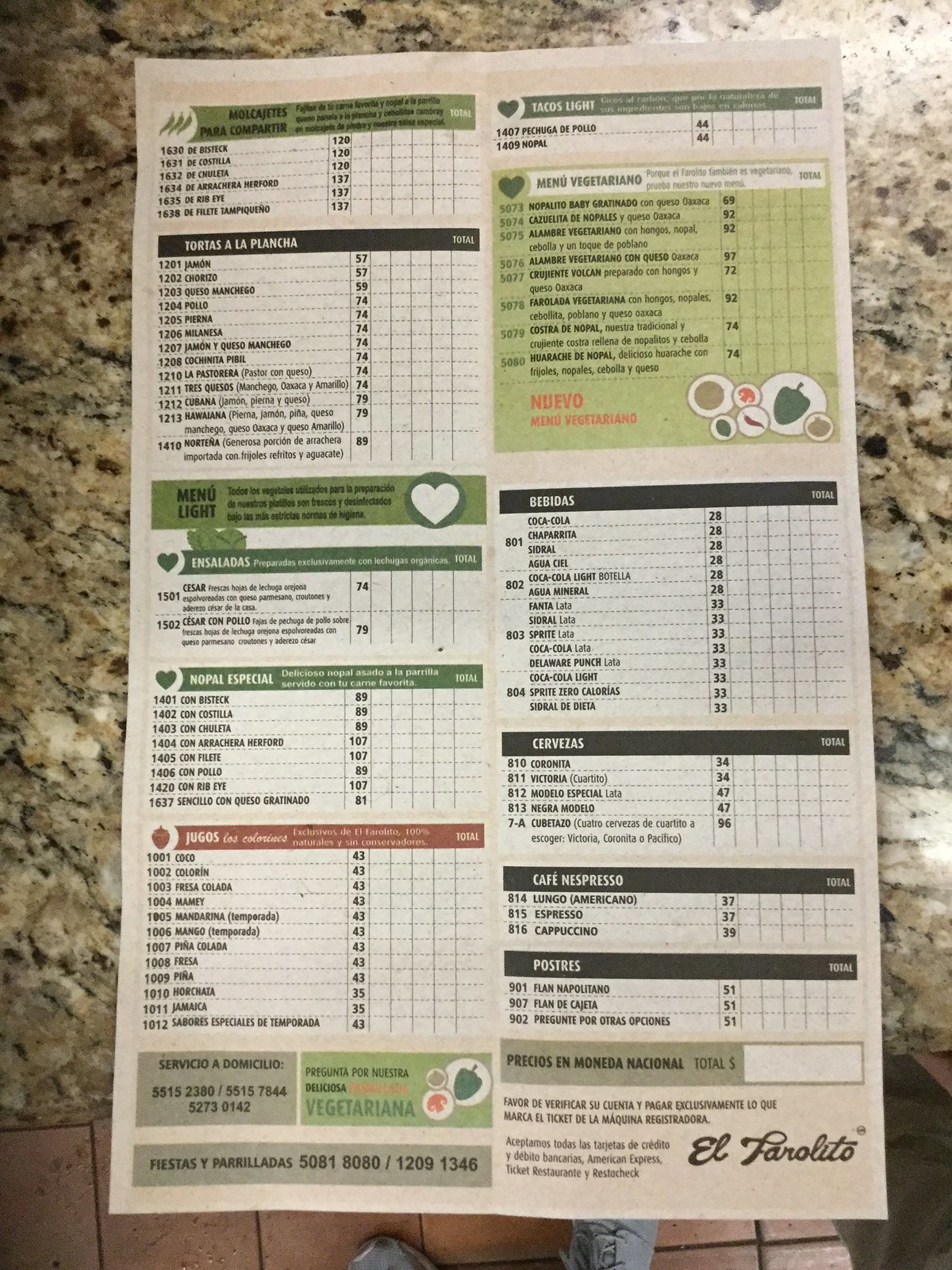### Descriptive Caption:

This image captures what appears to be a distant menu, challenging to read due to its distance. In the top left corner of the menu, a vibrant green section is visible, followed by approximately six rows of black text underneath it. Adjacent to this area, a long black rectangle contains noticeable white text at the end, spelling out "A-L-L-A-P-L-A-N-C-E-R." Below this segment, there are more rows displaying black text.

Progressing further down, another distinct section with a green background can be observed; it features a white heart icon. This area is succeeded by additional subcategories delineated with black text, detailing the items available for order.

On the right side of the menu, the top segment is shaded in a light green hue, accompanied by black text. This portion also showcases circular icons, each depicting different ingredients: one has a green pepper, another has a small eggplant, and yet another displays a red pepper. Continuing down the right side, there are more subcategories listed in black text.

Finally, in the lower right corner, elegant cursive writing spells out "E-L-F-A-R-O-L-I-T-S."